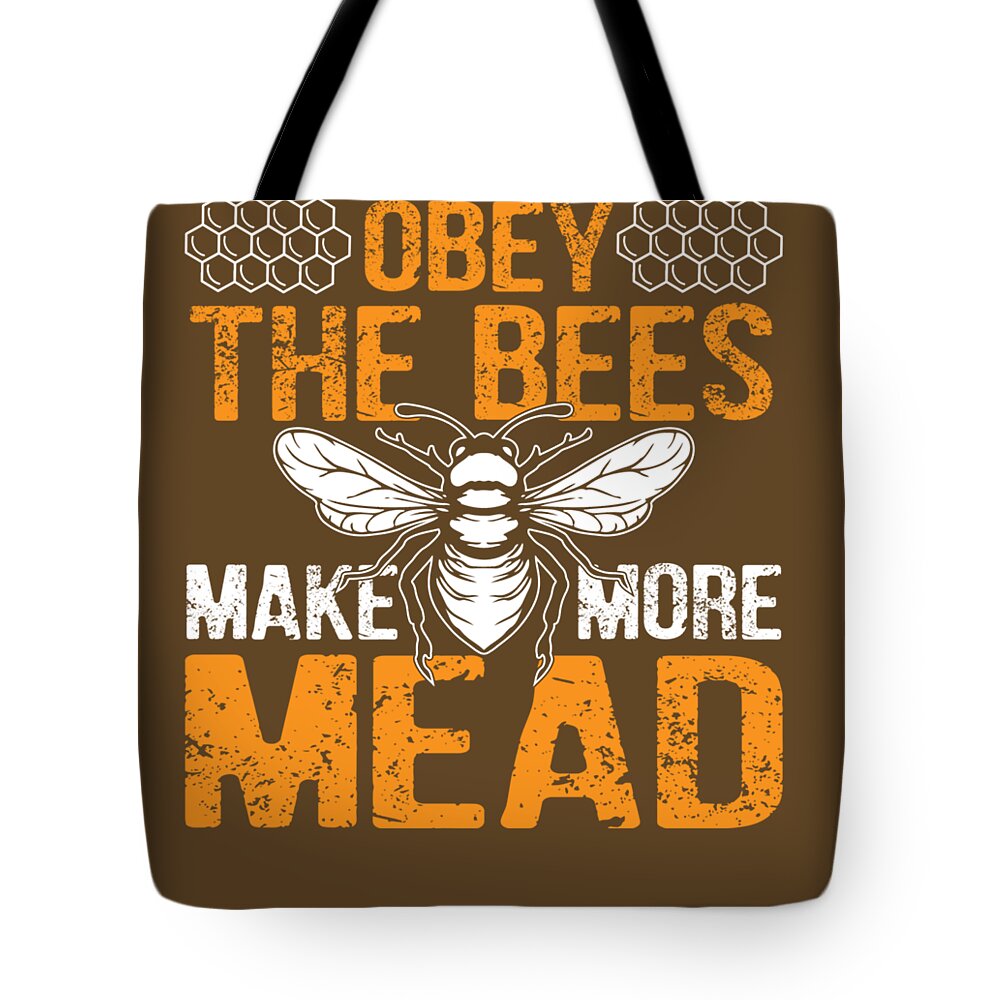The image features a square-shaped tote bag made of brown fabric with a black handle that appears cut off at the top. Across the top left and right corners, the bag displays white honeycomb shapes. In the center of the tote, bold, uppercase orange text with a grainy, speckled brown texture reads "OBEY THE BEES." The phrase "Make More" is positioned in white, also in an uppercase, distressed font. Below this, centering the design, is a large white silhouette of a bee with its wings spread. At the bottom of the tote, in the largest font size, the word "MEAD" appears in the same distressed orange text. The unique design of this tote bag juxtaposes rustic and bold elements to create an eye-catching accessory.